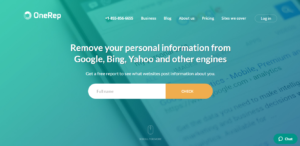The image is a small rectangular picture featuring a predominantly green and blue background. Within this backdrop, a tablet screen displays an internet browser. In the browser window, a white magnifying glass icon is visible inside a small blue square. The webpage contains a mix of blue and black text along with several white text sections layered on top.

In the top left corner of the screen, there is a white circle followed by the text "one rep" and adjacent blocks of white text. On the extreme right, there is an oval outlined with a thin white line that reads "log in." Below this, white text states, "Remove your personal information from Google, Bing, Yahoo, and other engines."

Beneath this phrase, a long white oval box, which appears to be a text input field, spans the width of the screen. Inside this white oval, some black text is discernible. The right end of the oval features an orange segment with white text that reads "check." Additionally, in the bottom-right corner is a small green oval with white text that says "chat," accompanied by a white text bubble icon.